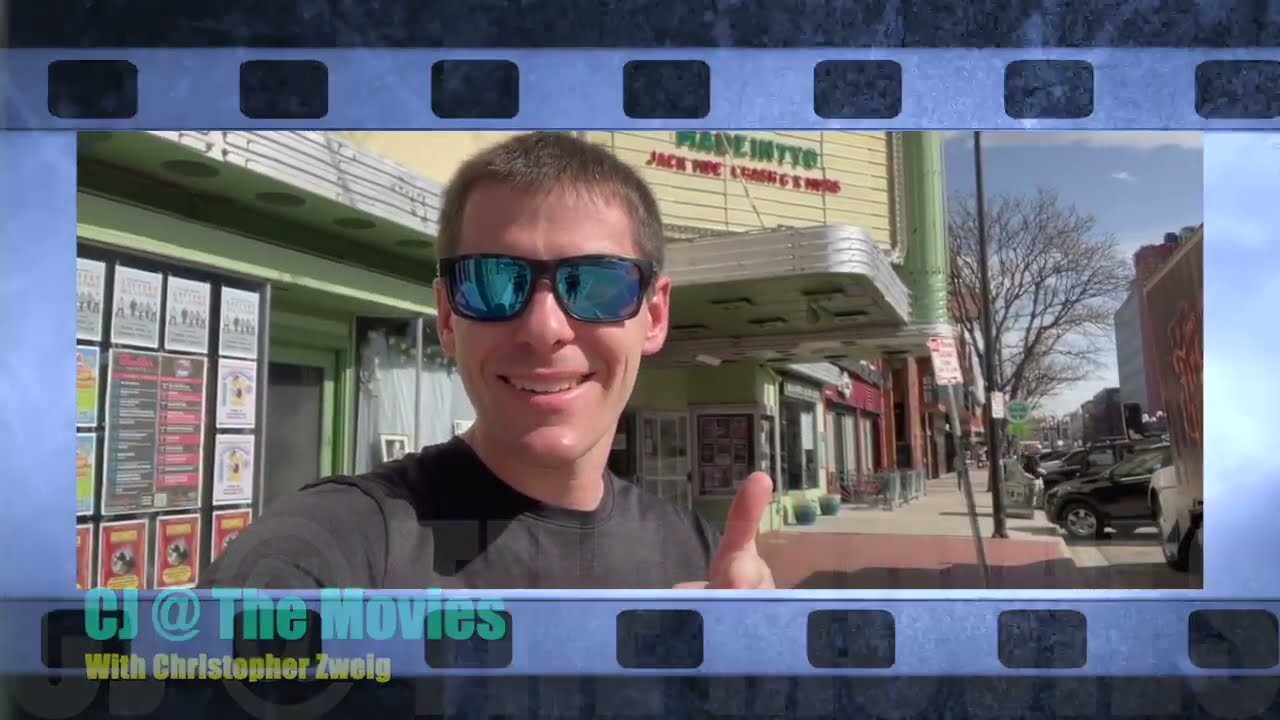In the image, a white man with light brown hair and a black short-sleeved shirt stands in front of a vintage movie theater, giving a thumbs-up with his left hand. He sports black sunglasses with blue reflective lenses and a cheerful smile. The movie theater behind him features a projecting awning with shiny aluminum trim and a green pole running up the middle. The marquee above, in cream color, displays unreadable text. Additional details include posters on the windows and walls and a paved brick walkway leading to the theater. In the distant background, there are parked cars, a leafless tree, a blue sky with white clouds, and other buildings. The entire scene is bordered by a dark and light blue filmstrip motif. In the bottom left corner, the caption "CJ at the Movies" appears in blue impact font, with "with Christopher ZWEIG" in yellow below it.